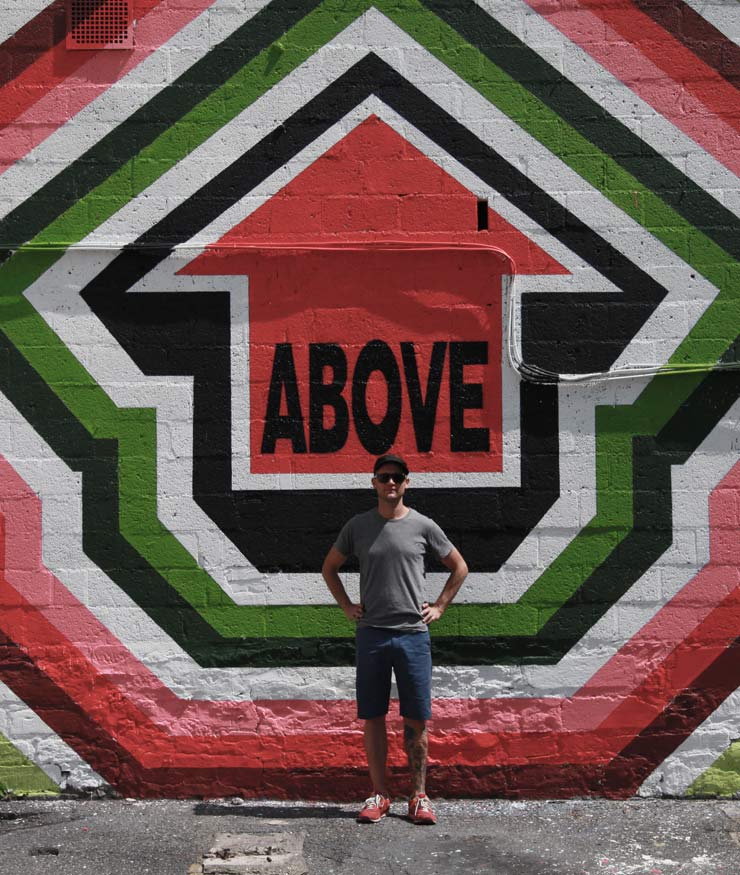In this vibrant and detailed outdoor image, we see a man standing in front of a cinder block wall painted with a large, intricate logo. The central feature of the mural is a bold red arrow pointing upwards with the word "Above" written in black letters on it. Surrounding the arrow are multiple layered borders in colors white, green, black, pink, maroon, creating a visually striking pattern. The man in the image is wearing a gray shirt, black hat paired with sunglasses, and blue shorts. His left leg is adorned with several tattoos, and he is wearing pink shoes with white laces. The ground beneath him is made of gray asphalt, scattered with stones, and it's illuminated by sunlight. In the upper left corner of the image, a red and pink vent is visible. There are also electrical wires running in a zigzag pattern across the wall. The man, possibly the artist behind the mural, stands proudly in this visually compelling and colorful scene.